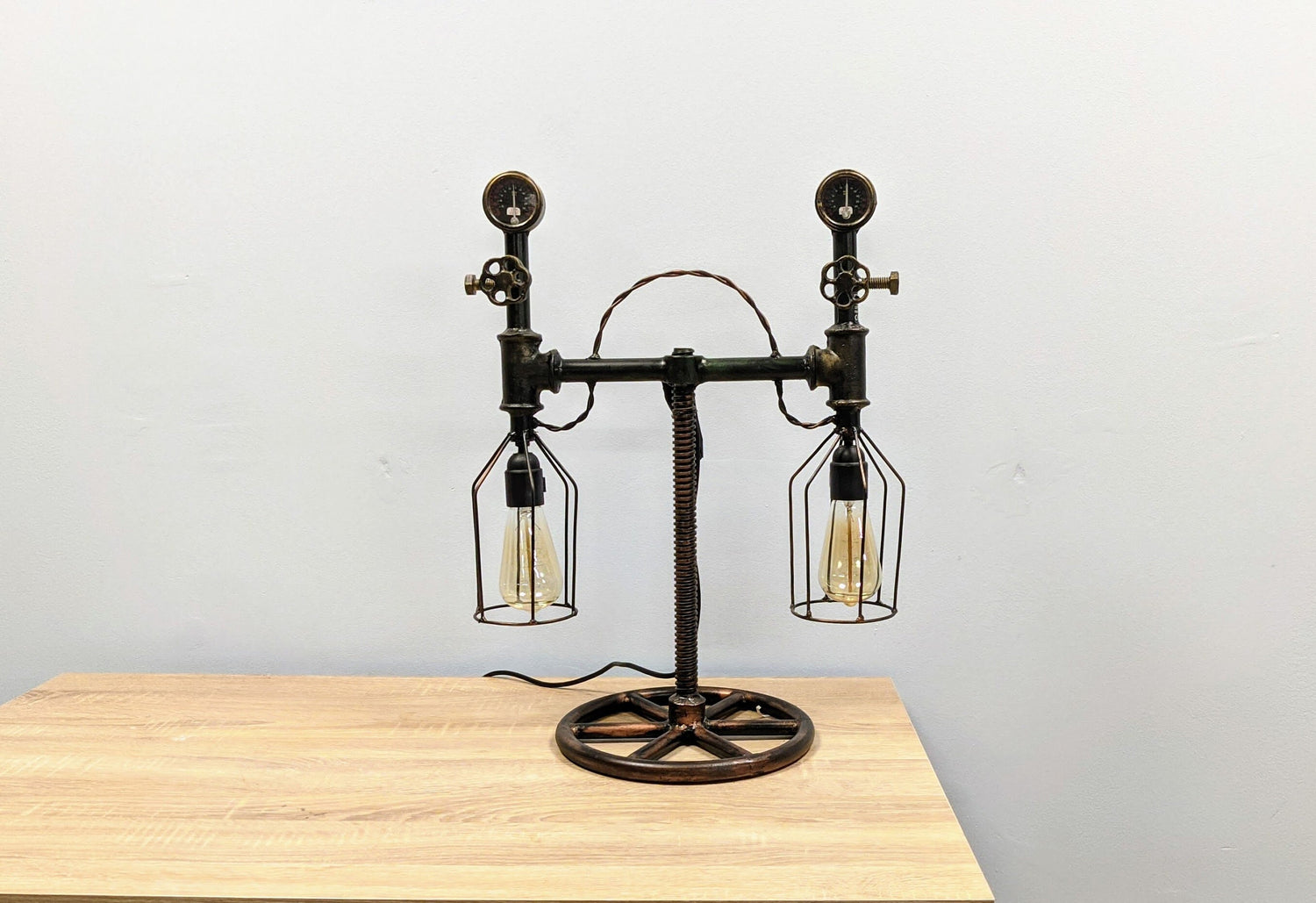The image portrays a custom-made lamp crafted from vintage machine parts, prominently set against a white wall and atop a pale-colored wooden table. The lamp's unique design features a sturdy base consisting of a metal spoked wheel. Rising from the center of this wheel is a large, ridged spring, which supports an H-shaped horizontal bar. At each end of this bar, there are intricate lamp assemblies adorned with Edison-style yellowed light bulbs, encased in protective metal cages. Each lamp assembly includes a valve wheel and a pressure gauge mounted above the valve, connected by a semi-looping metal line. Additionally, a power cable extends from the horizontal bar, trailing down beneath the table. The entire composition suggests an artistic blend of industrial elements and meticulous craftsmanship, creating a functional yet visually striking piece.